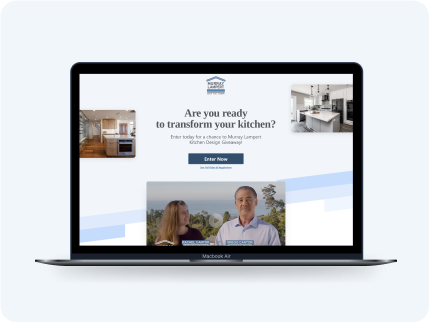The image portrays an advertisement for the MacBook Air. The focal point is the MacBook Air itself, illuminated on an elegant black and blue-bordered screen. Prominently displayed on the screen is the text "MacBook Air" at the bottom center. The computer's screen features a website or digital ad with the headline "Are you ready to transform your kitchen?" Below this headline, there's a call-to-action statement urging users to "Enter today for a chance to [blank, blank, blank, blank, blank]. Enter now."

The screen is sectioned into two main parts: to the right, three smaller images are displayed showcasing kitchen designs. The first image captures a modern kitchen with white countertops and black appliances. The second image shows a kitchen with hardwood floors and wooden cabinets, with what appears to be a stove integrated into the cabinetry.

Below the call-to-action statement, there's a video thumbnail featuring a young woman with long brown hair and an older Caucasian man dressed in a buttoned-up shirt. A play button centered on the video thumbnail suggests it's clickable for playback. Underneath the video, likely in blue text, are their names, providing a personal touch to the advertisement.

This detailed visual experience not only highlights the elegance of the MacBook Air but also integrates a dynamic and interactive kitchen remodeling promotion.